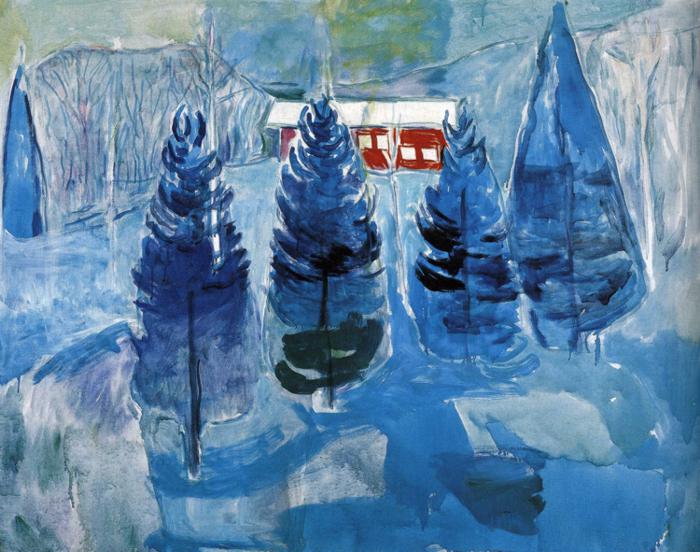This painting, done in a primitive, abstract style, presents a joyful yet serene winter scene dominated by shades of blue and white. In the foreground, four prominent blue pine trees, narrow at the bottom and pointier at the top, stand like sentinels. Each tree is detailed with dark accents, suggesting depth and shadow. The ground, rendered in lighter blues and whites, evokes a snowy landscape where the snow in front of the trees is lighter, contrasting with the darker shadows behind them.

At the center of the scene, a glossy, ice-like blue pond captures reflected light, adding a sense of cold stillness. Behind the trees, a low, long red house with a snow-covered white roof stands out vibrantly. This house features four visible windows, while one side remains partially hidden by the trees. The background reveals a less defined grove of trees, suggesting a dense, frozen forest receding into the distance.

Up above, the sky is an indistinct blend of whites and lighter tones, with a subtle touch of yellow on the left side, hinting at either sunrise or sunset. The overall composition is rich with beautiful shades of blue, white, and a striking red, encapsulating the tranquil beauty of a winter’s day.